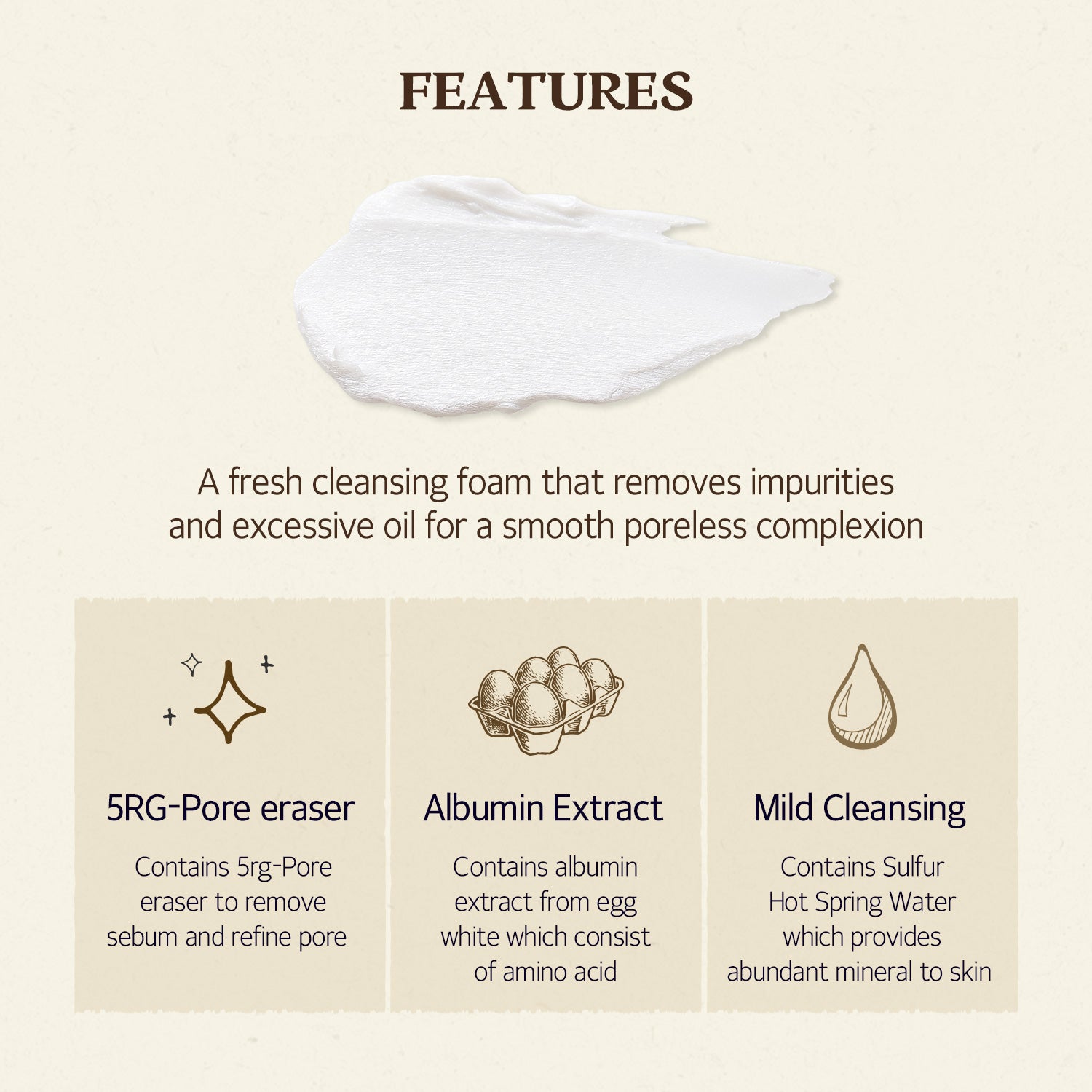The advertisement is for a fresh cleansing foam designed to remove impurities and excessive oil for a smooth, poreless complexion. The background is a soothing, very light beige or tan color, almost resembling organic cotton or linen, with dark brown lettering. At the top, in all capital letters, it says "FEATURES," with a white smear of what looks like shaving or face cream stretching from left to right underneath the word.

Below this, there are three distinct panels, each with additional information about the product’s features, outlined in slightly darker tan text boxes. 

1. The first panel on the left has a black text on a dark tan background and features a small hand-drawn star shape. It reads: "5RG Pore Eraser: contains 5RG pore eraser to remove sebum and refine pores."
2. The center panel depicts an open carton of six eggs and states: "Albumin Extract: contains albumin extract from egg white, which consists of amino acids."
3. The third panel on the right shows a large moisture droplet and notes: "Mild Cleansing: contains sulfur hot spring water, which provides abundant minerals to the skin."

This detailed layout gives a comprehensive look at the key ingredients and benefits of the cleansing foam, with emphasis on its organic and mineral-rich components.